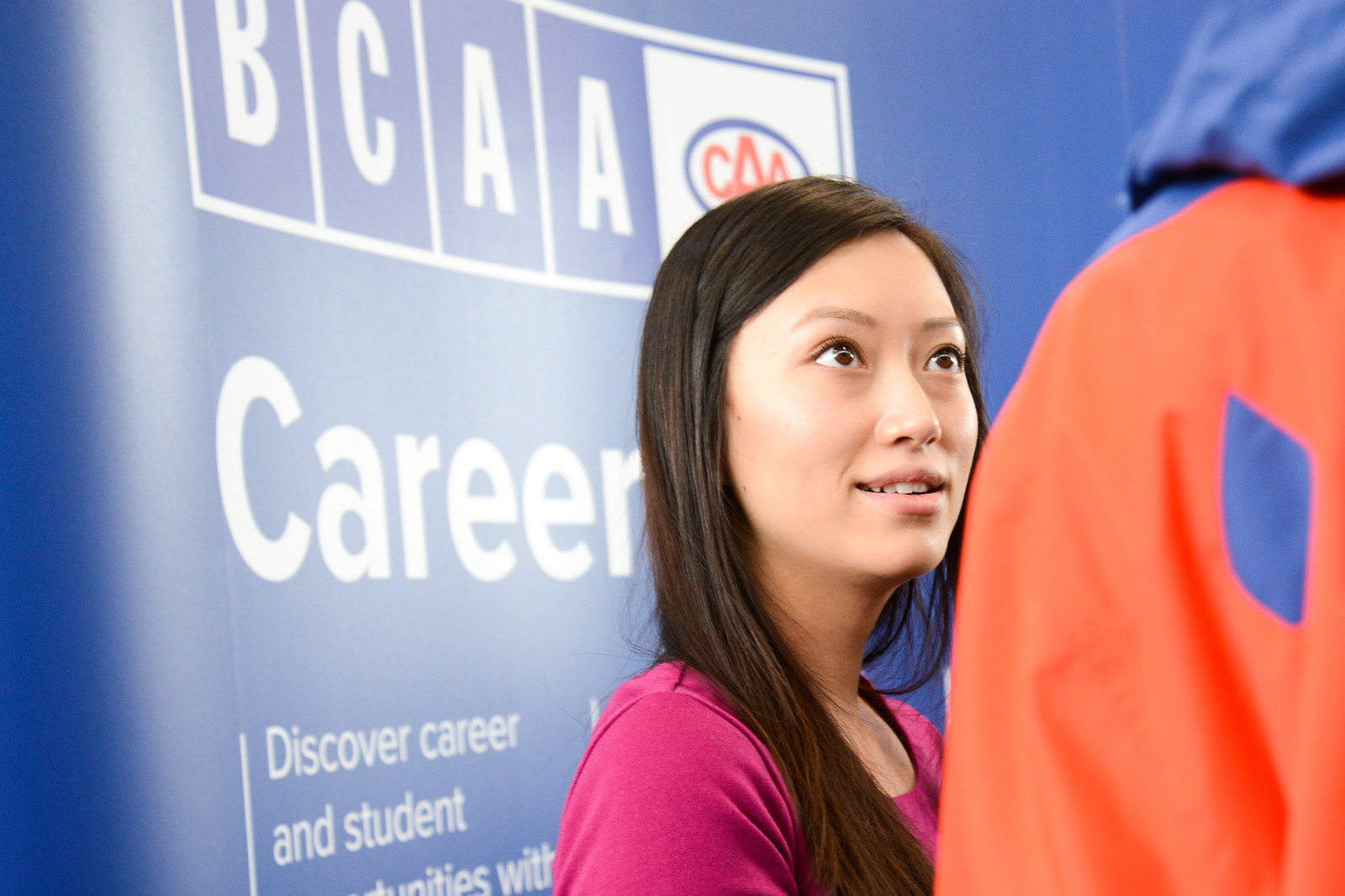The image depicts a young, Asian woman with long black hair and brown eyes, engaged in an intense conversation while looking up at someone wearing an orange and blue coat whose face is not visible. She appears to be in her early 20s and is centered in the middle of the frame. Her mouth is slightly open, suggesting she's listening attentively, and she is dressed in a pink shirt. Behind her is a blue backdrop featuring the BCAA logo at the top, characterized by bold white lettering. Below the logo, the word "career" is prominently displayed along with additional text that reads "discover career and student," partially obscured by her presence. This scene might be set at a booth in a career fair or convention, indicated by the backdrop and context clues.